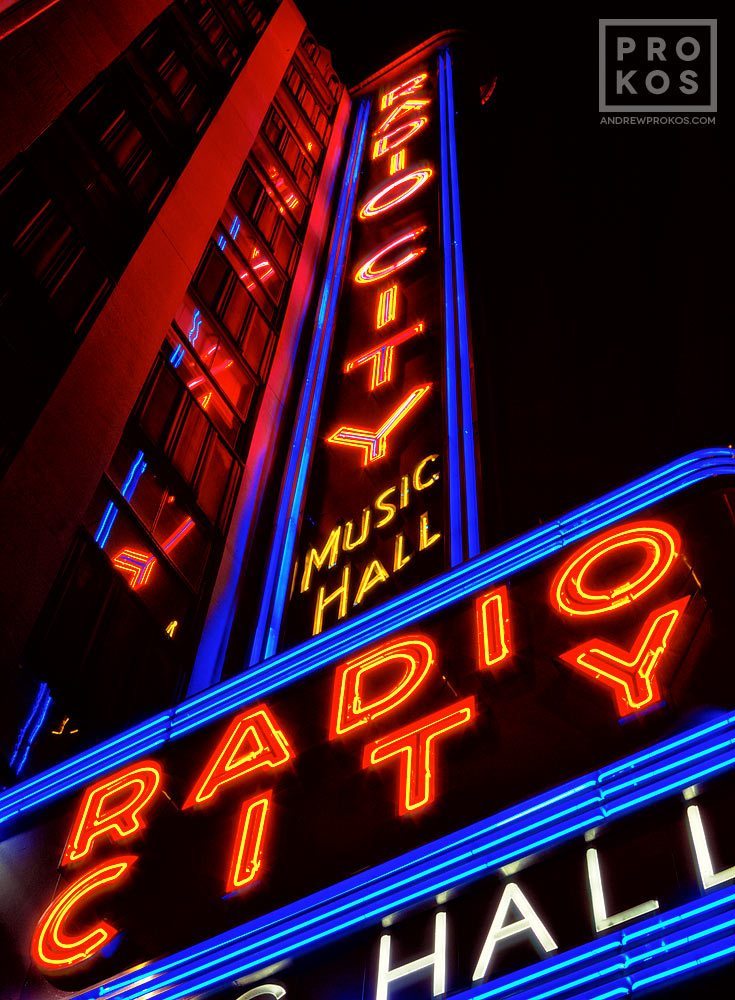This vertically-aligned rectangular image captures the iconic Radio City Music Hall sign at night, against a solid black background. The photograph, taken from the ground looking upward at an angle, showcases the sign against the backdrop of a multi-story building, which appears partially visible on the left upper corner. The building, difficult to fully discern but estimated to have around 10 stories, has illuminated windows and brown stone between the window panes.

The centerpiece of the image is the narrow rectangular sign descending from the top. This sign features the words "Radio City" printed vertically in vibrant red or orange neon letters, bordered by blue neon tubes on each side. At the very bottom of the vertical sign, "Music Hall" appears in yellow letters. Additionally, the image captures another part of the sign where "Radio City" is printed horizontally but at an angle from the lower left to the middle right, also featuring blue neon borders. Below this horizontal section, the word "HALL" is visible in all caps with white letters, though the full text before it is cut off.

At the top right corner of the image, there is a gray box containing the text "Pro KOS Entertainment Group" or "ProKost.com" in white letters. This adds a final touch of detail, visible against the dark background of the nighttime scene. Overall, the image provides a detailed and vivid depiction of the Radio City Music Hall sign, with its neon lights reflecting off the building's windows.